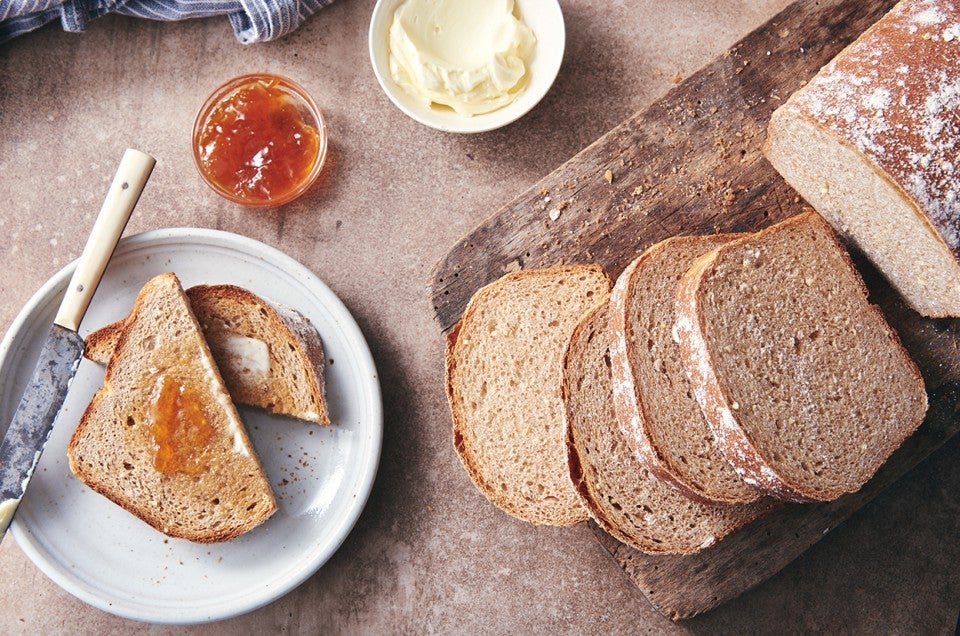This image captures a breakfast table scene showcasing a rustic, fresh-baked loaf of rye bread with a light dusting of flour, set on a wooden butcher block. The loaf, partially sliced, reveals four neatly cut pieces aligned at the front of the board. To the left side of the scene, a white plate holds two triangular slices of toast; one adorned with both butter and jam, and the other with just butter. Accompanying the plate is a knife with a white handle, evidently used for spreading the condiments. Adjacent to the main setup are small bowls containing butter and jam— the jam in a glass bowl and the butter in a plastic one—completing the wholesome breakfast preparation.